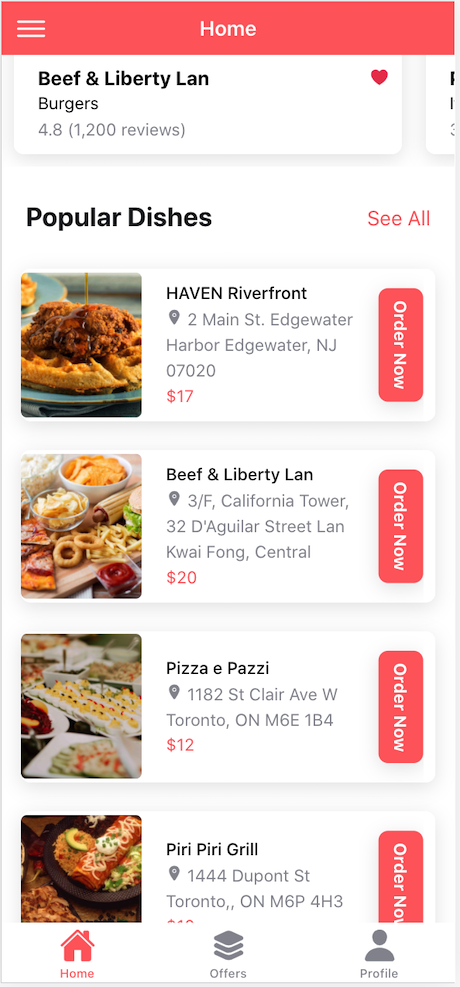The image showcases a vibrant mobile app with a salmon and white color scheme, designed for a food delivery service. At the top of the screen, a favorited dish, "Beef and Liberty Land Burgers," is prominently displayed. Below this, the section titled "Popular Dishes" features an option to explore more dishes. Each meal listed has an "Order Now" button, indicating that users can place orders directly through the app. The locations of the available dishes span the globe, including Kwai Fong Central, Harbor Edgewater in New Jersey, and Toronto, Ontario. The listed dishes include Haven Riverfront, Beef and Liberty Land, Pizza e Pazzi, and Piri Piri Grill, showcasing a diverse range of culinary options.